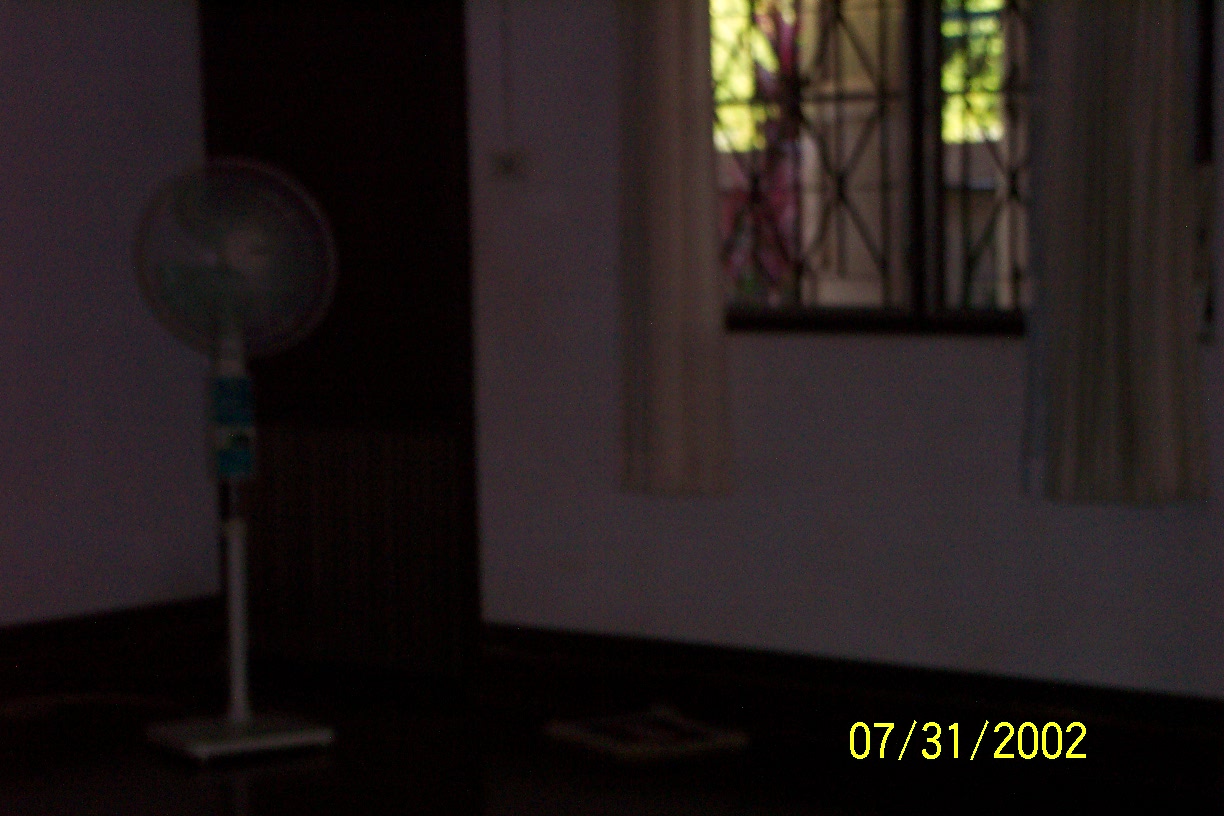The image depicts the interior of a possibly living room setting. Prominently featured is a window adorned with decorative bars on the exterior, flanked by two white curtains. The walls in the room are white, and there is a dark-colored door, seeming to provide access to an outdoor porch. The floor appears to be made of wood. On the left side of the image stands a tall, white pedestal lamp. The bottom right-hand corner of the image shows the date "07-31-2002", indicating the photograph was taken on July 31, 2002.